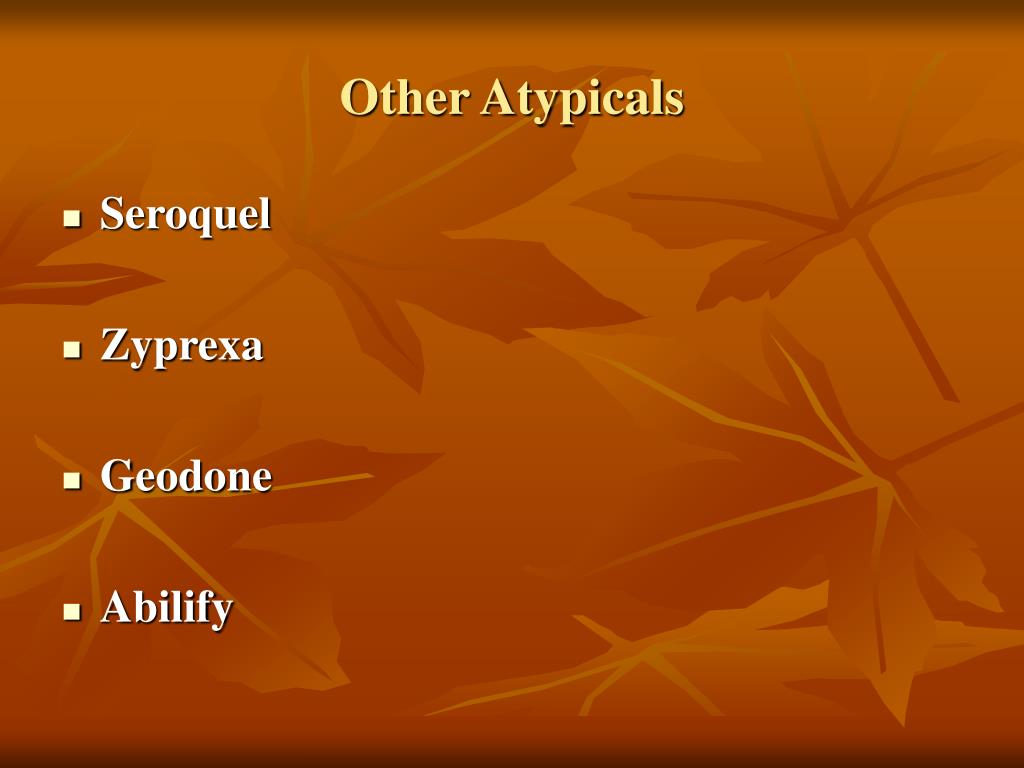The image appears to be a PowerPoint slide with a square-shaped layout. The overall background is a medium brown color featuring a design of autumn leaves in slightly darker and lighter shades of brown, blending seamlessly across the surface. On the left side of the slide, there are four yellow bullet points, each with the following names in white text: Seroquel, Zyprexa, Geodon, and Abilify. The title, "Other Atypicals," is prominently displayed in yellow letters at the top center of the page, with an initial capital letter for each word. The slide is bordered on the top and bottom with a slightly darker brown horizontal line, while the sides are left without borders. The leaves in the background have visible stems and spines, adding texture to the design. The background color might also incorporate subtle hues of orange. The text is formatted in a basic sans-serif font and is left-aligned for the bullet points.